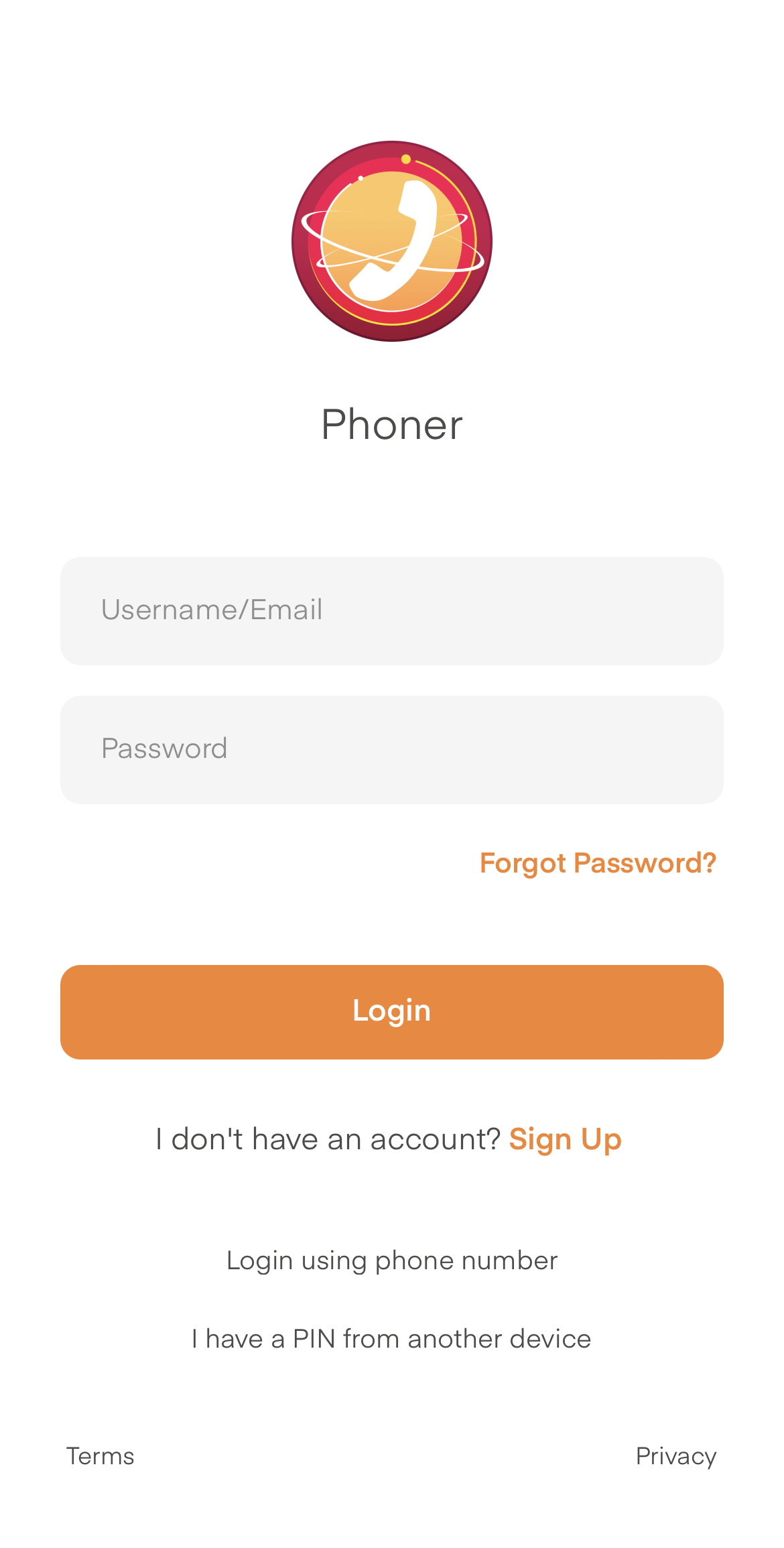This image is a screenshot of a login form, presented in portrait mode, with a predominantly white background. At the upper center of the form, there is a logo consisting of a white phone icon inside a yellow circle, encircled by global lines, all enclosed within a red border with an additional orange outline, and ultimately surrounded by a red circle. Beneath the logo, the word "Phoner" is displayed in capital letters.

The form comprises several sections for user input. The first field prompts for a "Username or email," followed by a "Password" field. To the right of the password field, an orange-colored live link option labeled "Forgot password" allows users to retrieve their password.

Below these fields, there is an oversized orange button with the word "Login" in small white font, leading to a significant amount of unused space on the button.

Following the login button, there is a statement, "I don’t have an account?" with an unnecessary question mark, after which there is an orange live link labeled "Sign up" for new users to create an account.

Additional options include "Login using phone numbers" and "I have a pin from another device." At the bottom, the text "terms" and "privacy" appear on the left and right sides, respectively, likely as live links but not highlighted in blue, deviating from the traditional link format.